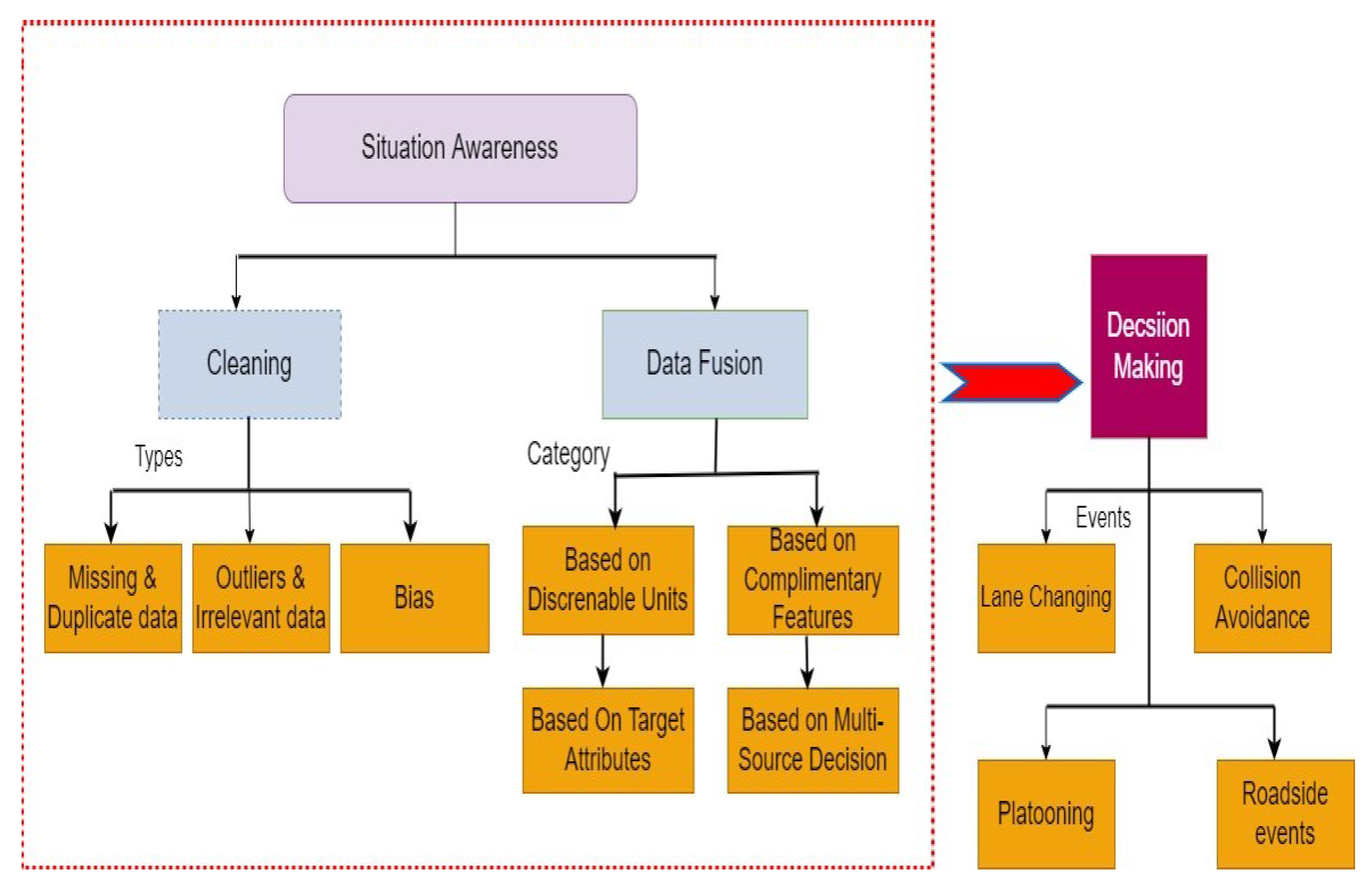The image depicts two interconnected flowcharts, or decision trees, emphasized by a red dotted outline and a red arrow. The larger flowchart on the left, enclosed within a red dotted square, begins with a light purple rectangle labeled "Situational Awareness." This branches into two gray boxes: "Cleaning" and "Data Fusion." The "Cleaning" box further branches into three orange boxes, labeled "Missing and Duplicate Data," "Outliers and Irrelevant Data," and "Bias." The "Data Fusion" box splits into four orange boxes: "Based on Discernible Units," "Based on Complementary Features," "Based on Target Attributes," and "Based on Multisource Decision."

To the right, a red arrow points from the larger flowchart to a smaller one, beginning with a purple rectangle labeled "Decision Making," though the word "Decision" is misspelled. This smaller flowchart branches into two orange boxes, "Lane Changing" and "Collision Avoidance." Each of these branches further into one additional orange box, labeled "Platooning" and "Roadside Events," respectively. This detailed flowchart illustration showcases the hierarchical decision-making processes involved in situational awareness and subsequent actions.